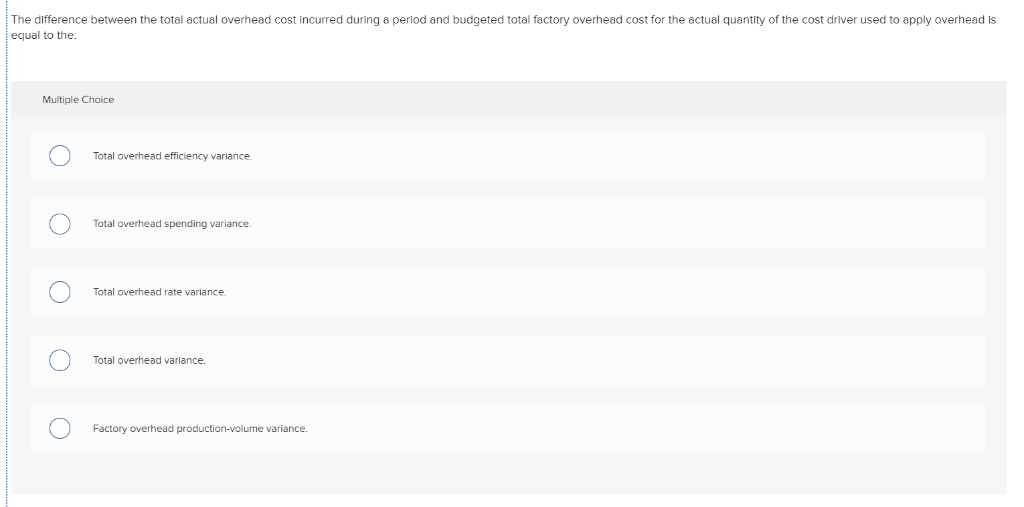This image depicts a screenshot of a website displaying a multiple choice exam question. The page has a white background and features a light gray header labeled in black text as "Multiple Choice." Below the header, the question is presented in black text: "The difference between the total actual overhead cost incurred during a period and budgeted total factory overhead cost for the actual quantity of the cost driver used to apply overhead is equal to the?" The possible answers are displayed in individual white bars that do not extend to the edges of the gray box, creating gray spaces between each white bar. On the left side of each bar, there is a round blue circle, and the respective answers are written in black lettering within the bars. There are five answer options: 
1. Total overhead efficiency variance
2. Total overhead spending variance
3. Total overhead rate variance
4. Total overhead variance
5. Factory overhead production volume variance

A blue line runs vertically along the left side of the entire page, adding a subtle visual separator.